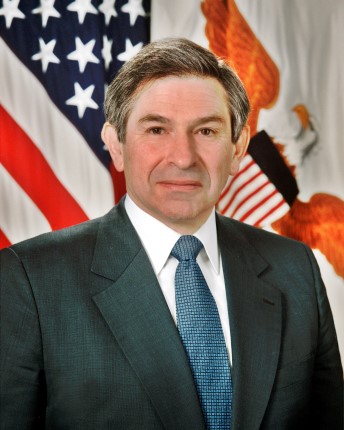This portrait features Paul Wolfowitz, an older Caucasian man, possibly in his 40s or 50s, seated and visible from the chest up. He is positioned against a backdrop of two flags: the American flag with its red and white stripes and blue field of white stars on his left, and a state flag on his right. The state flag has a white background and prominently displays an eagle with orange wings and a shield on its chest, which is striped in red and white. Wolfowitz wears a dark gray suit complemented by a white collared shirt and a blue tie. His hair is a salt-and-pepper mix, more salt than pepper, and parted neatly over his raised eyebrows. He gazes directly at the viewer with a blank expression, neither smiling nor frowning, giving the impression of a professional headshot.